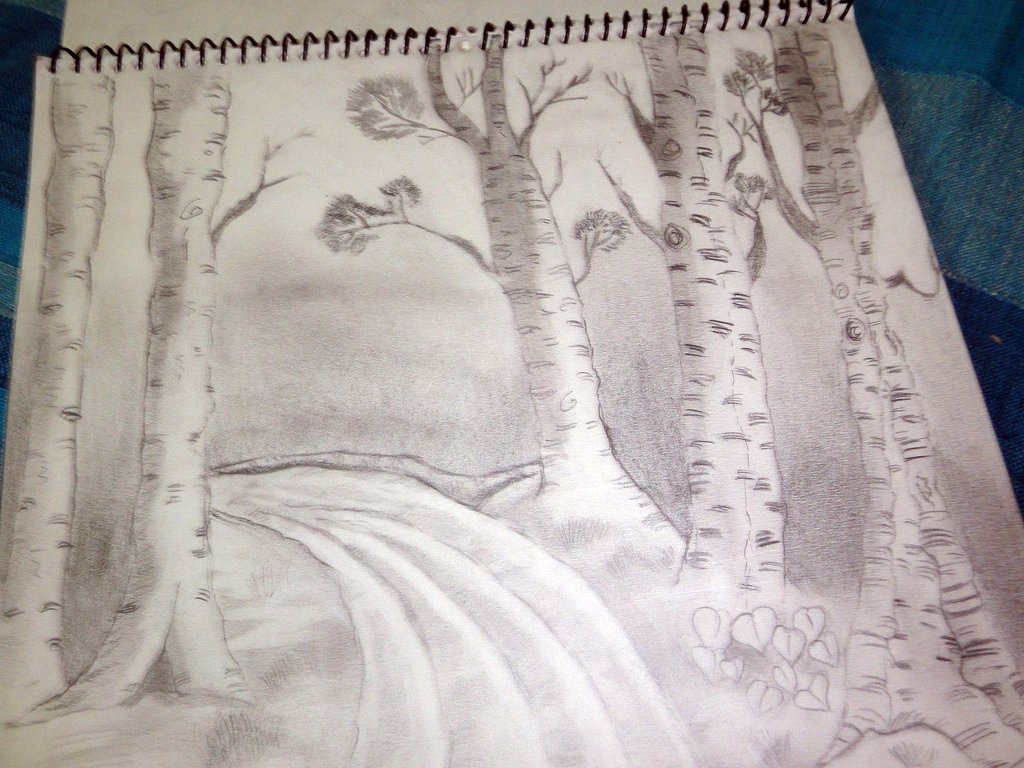A detailed hand-drawn pencil sketch depicts a forest of bare oak trees, with leaves starting to fall. The artist employs significant shading to create depth and texture, capturing the transition of seasons. In the foreground, a roadway or path winds through the forest, possibly suggesting snow tracks, hinting at a wintery setting. The drawing, while amateur, showcases an earnest effort and a keen eye for detail. The sketchbook rests on what appears to be a bed or bedsheets, and the photo is taken in landscape orientation.